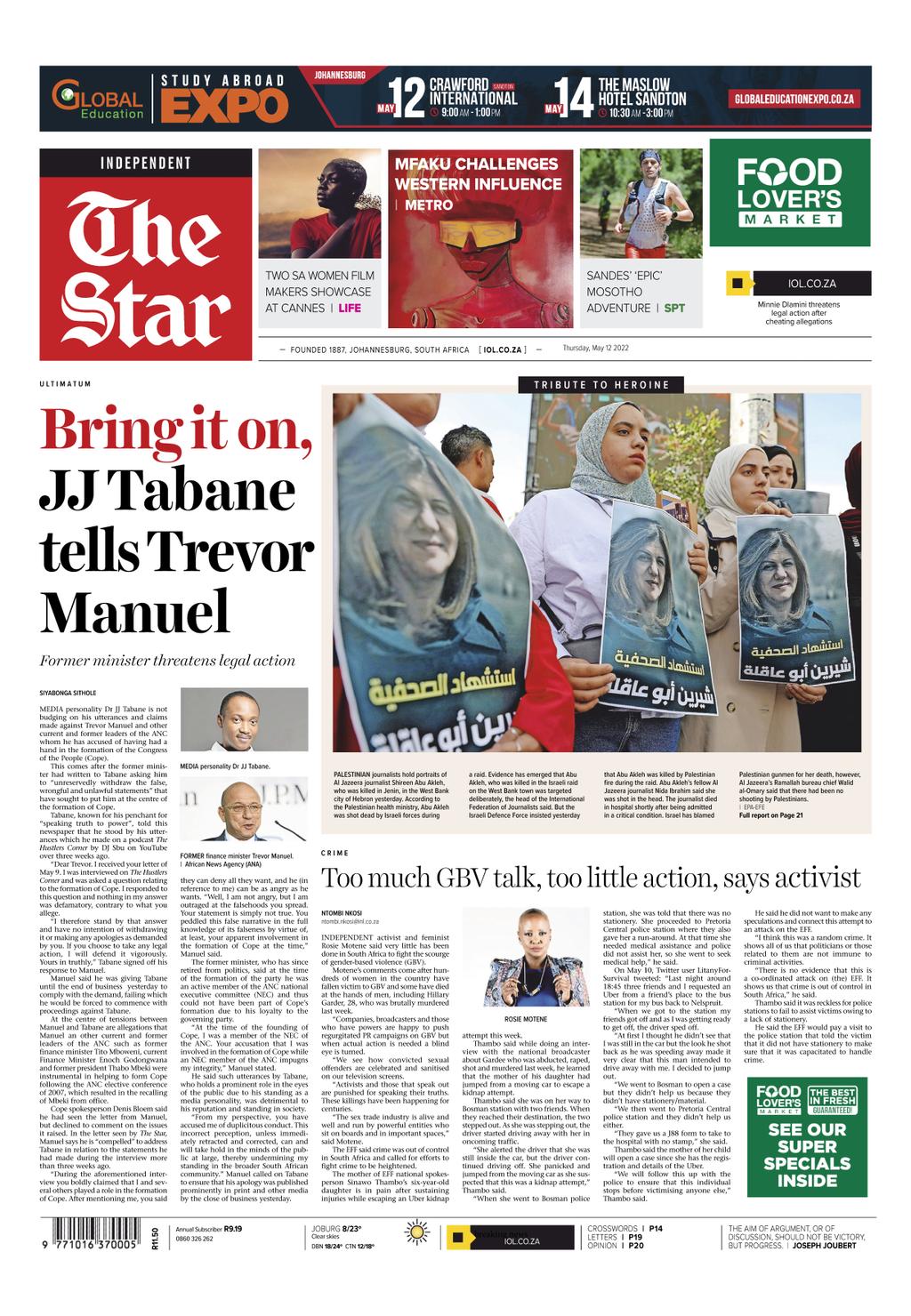This image is a colorful, detailed screenshot of a newspaper front page. Dominating the page are several striking headlines, such as "Bring it On: J.J. Tobain Tells Trevor Manuel" with a subhead indicating that the former minister is threatening legal action. Another prominent headline reads, "Too Much J.B.V. Talk, Too Little Action, Say Activists." 

The page features a barcode in the bottom left corner and a small sun graphic, likely indicating the weather forecast. On the right side, there’s a bold advertisement in green and white text that reads, "Food Lovers, Your Super Specials Inside—The Best and Fresh."

In the lower section, a headline reads "Tribute to Heroine," accompanied by three photographs of a short-haired woman. Some of the text appears in a language other than English and is not easily decipherable. 

At the top left, the newspaper is identified as "Independent" and "The Star," with a related headline announcing, "Two SA Women Filmmakers Showcase at Cannes." Another "Food Lovers Market" promo is visible in the top right. The central image features a woman with possible Arabic writing on it, surrounded by various other pieces of text and smaller images, creating a dense and information-rich front page.